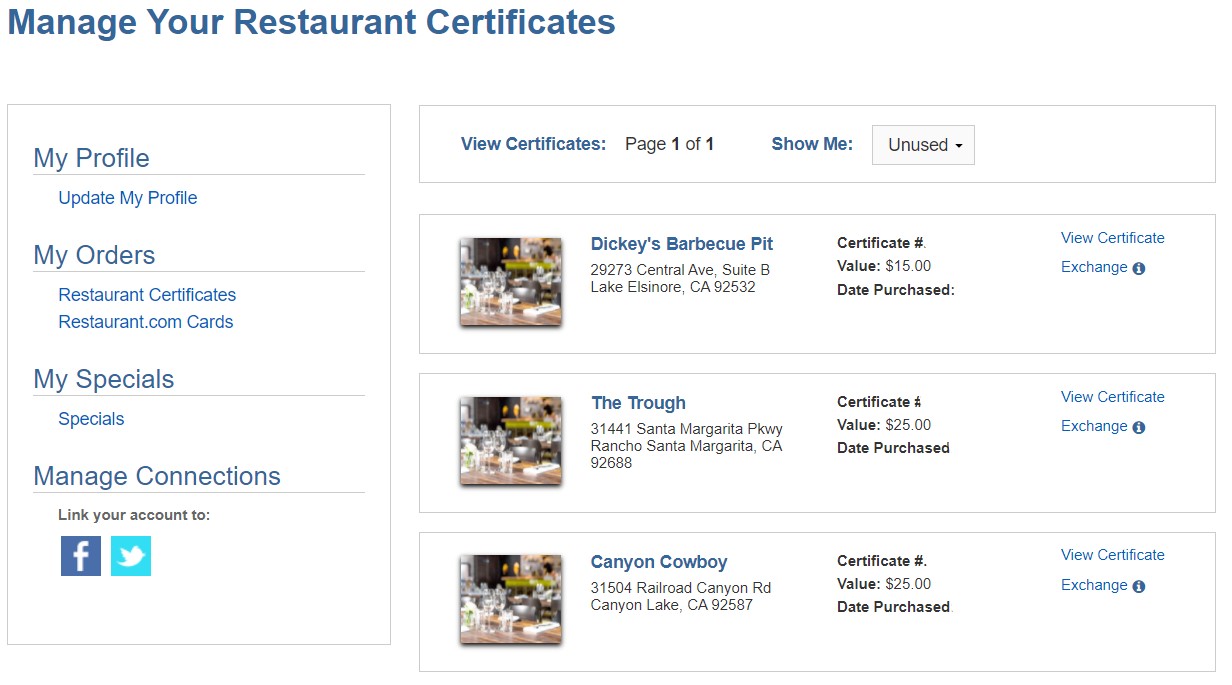This screenshot depicts a restaurant management webpage on restaurant.com. The interface shows a blend of navigation options and featured restaurants. 

To the top left, a header in dark blue text states, "Manage Your Restaurant Certificates." Below this, the left sidebar displays several sections starting with "My Profile" in a prominent font, followed by "Update My Profile" in smaller blue text. The next main section, in large blue text, labeled "My Orders" leads into a list of subsections: "Restaurant Certificates" and "Restaurant.com Cards." Further down, the sidebar lists "My Specials," followed by "Manage Connections," which includes links to "Facebook" and "Twitter," represented by their respective logos, indicating social media integration options.

On the right side of the screenshot, a section highlights featured restaurants. At the top is "Dickies Barbecue Pit," followed by "The Trowel" and "The Canyon Cowboy." Interestingly, all restaurants share the same generic image, suggesting placeholder or uncustomized visuals. This design and some elements appear outdated, hinting at the screenshot's older origin.